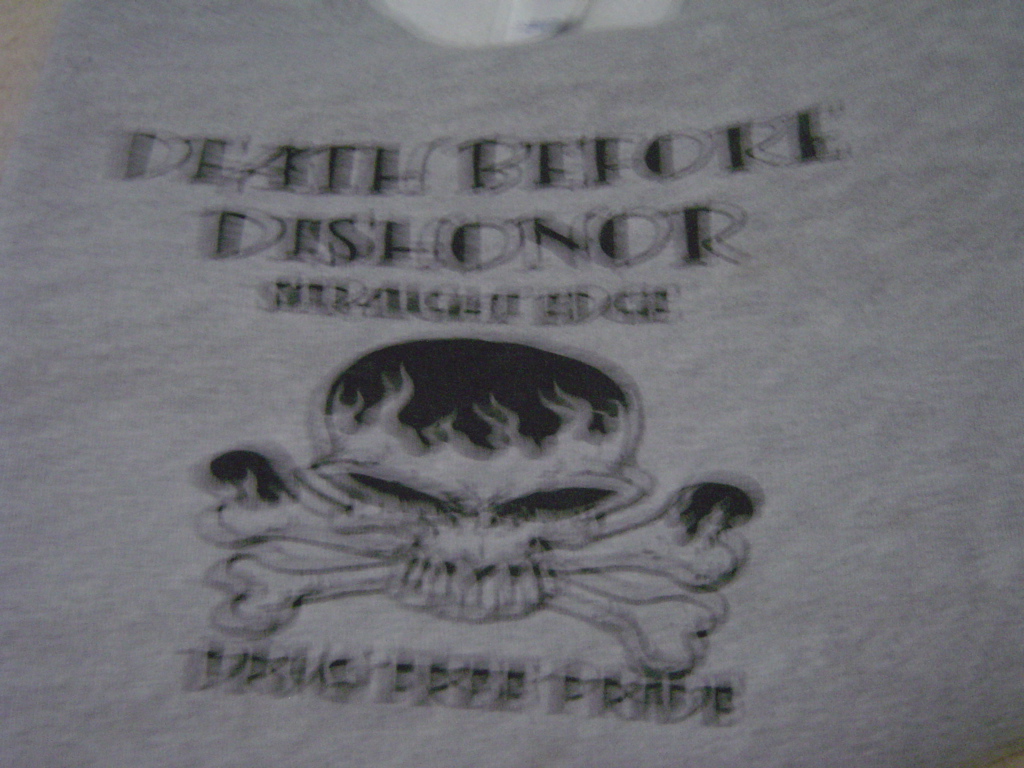The image depicts a close-up of a gray t-shirt adorned with a bold black design. Prominently featured in black lettering are the words "Death Before Dishonor," suggesting a theme inspired by military or Marine principles. At the center of the design is an imposing skull with flames emanating from its eyebrows, giving it an angry expression. Behind the skull, two bones are crossed in an X formation, adding to the menacing appearance. Below this graphic, there is additional text, although it's difficult to discern clearly due to the close-up nature and blurriness of the image. It appears to reference a phrase like "Drug Free Parade," indicating that the t-shirt may be promoting a motivational or anti-drug message. The overall impression is one of strong, assertive imagery, likely intended to inspire or convey a strong principle or message.